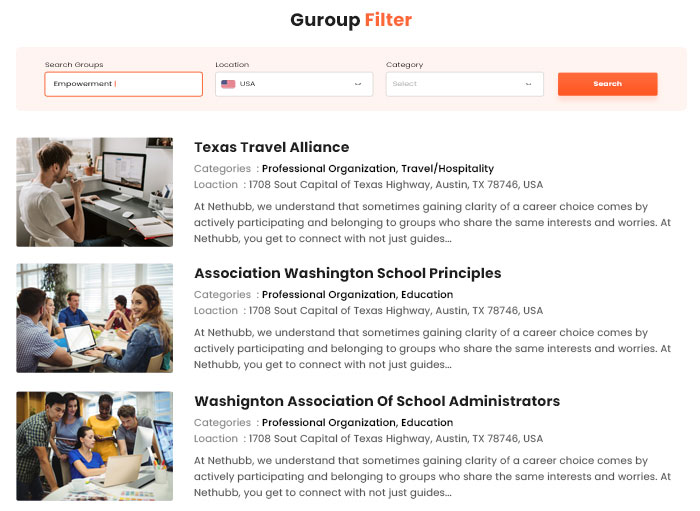Certainly! Here's a cleaned-up and detailed caption for the image:

---

This screenshot appears to capture a web page titled "Gurope Filter," prominently displayed at the top center with "Gurope" in black text and "Filter" in orange. Directly below this title, there is a reddish-orange box divided into several sections: a field for "Search Groups," a drop-down menu for "Location," a search bar labeled "Category," and a bright orange "Search" button on the far right.

Underneath this search section, the page is divided into three distinct sections, each following a consistent format. On the left side of each section, there is a photograph:

1. The first section features an image of a person looking at a computer screen. The headline reads "Texas Travel Alliance," categorized under "Professional Organization - Travel & Hospitality."
   
2. The second section displays an image of people sitting around a table, with a woman smiling in front of her laptop. The headline here is "Association Washington School Principals," categorized under "Professional Organization - Education."
   
3. The third section includes a photograph of a woman behind a computer, with four other people behind her, staring at the screen. The headline for this section is "Washington Association of School Administrators," again categorized under "Professional Organization - Education."

Each of these sections includes additional information on the location and a brief description of the respective organization.

---